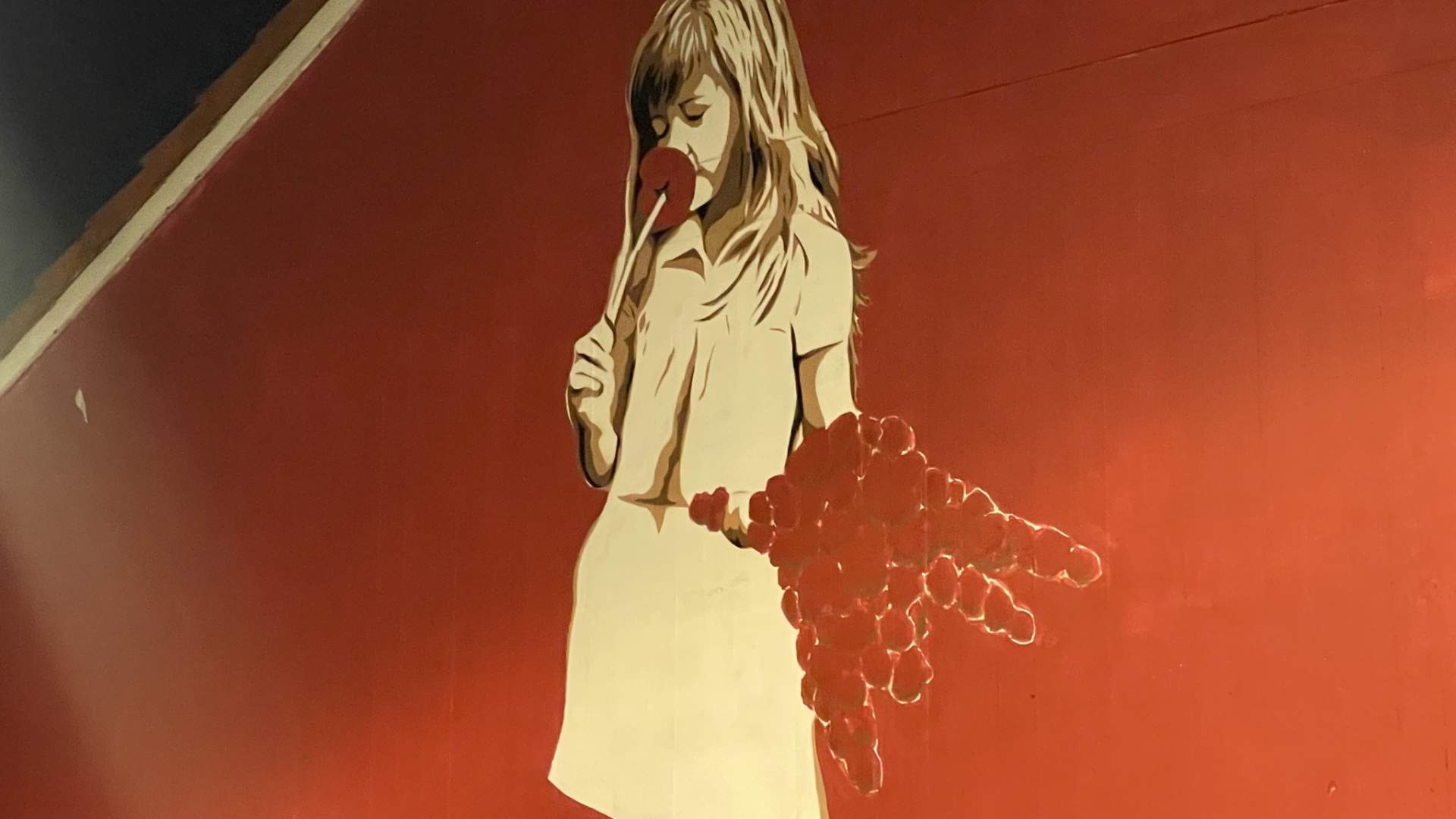This detailed painting on a smooth red background features a little girl with long blonde hair and short bangs, captured in an amber and white, film-negative-like coloration. The girl is depicted in a collared, short-sleeved dress that buttons down the front. She is intently smelling a red poppy that she holds in her right hand, while her left hand grasps a large bouquet of similar poppies. The painting is bordered by a thin white line and framed with wood, noticeable in the upper left corner. The girl's eyes are closed, highlighting her focus on the flower. Despite the predominantly red background, there is a small section of blue in the top left, separated by a white diagonal line, giving it a dynamic, layered appearance indicative of spray paint art.